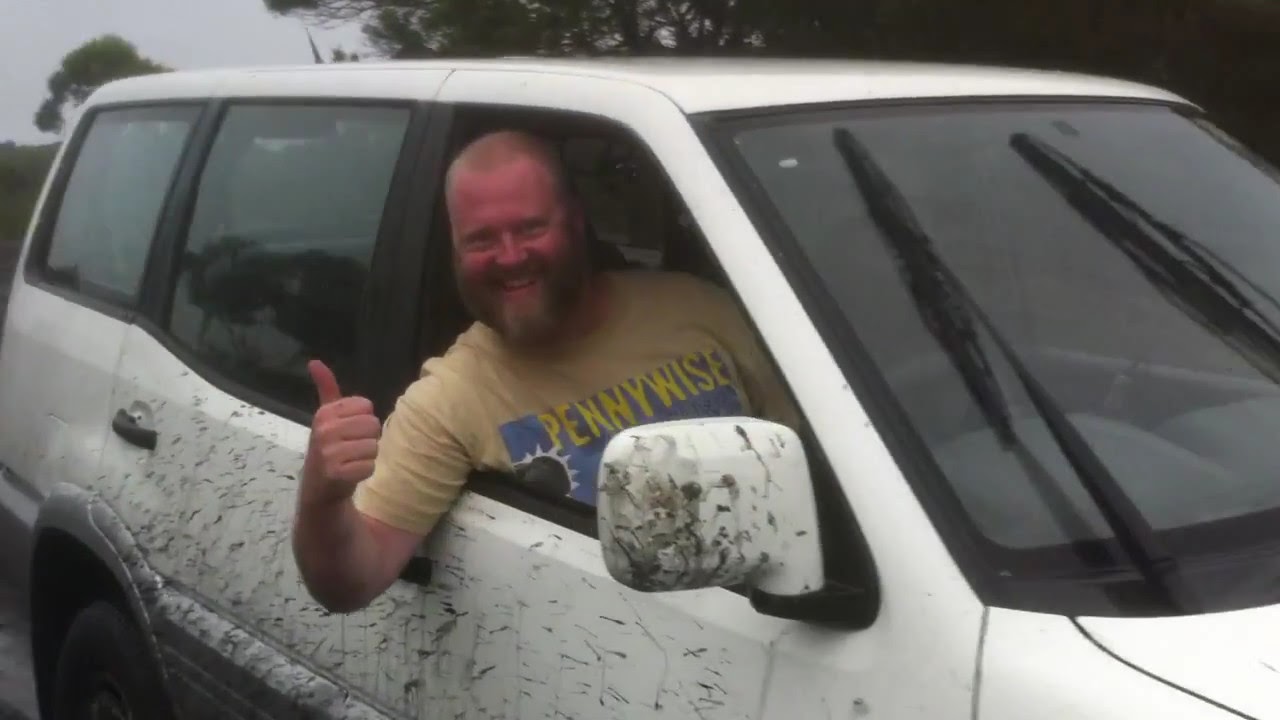A Caucasian man with a full beard and short, light brown hair leans out of the passenger side window of a white, mud-splattered SUV, smiling broadly and giving a thumbs up to the camera. He is wearing a light yellow short-sleeved shirt featuring the word "Pennywise" in bright yellow letters across the chest, underneath which is a blue square. The vehicle, an SUV with windshield wipers standing upright, suggests it might have recently rained or is currently overcast. Mud streaks cover the right-hand side of the SUV, including the side mirror and doors. In the background, a gray, cloudy sky is visible, along with a few trees. The setting appears to be outdoors, giving a slightly rugged and weathered feel to the scene.